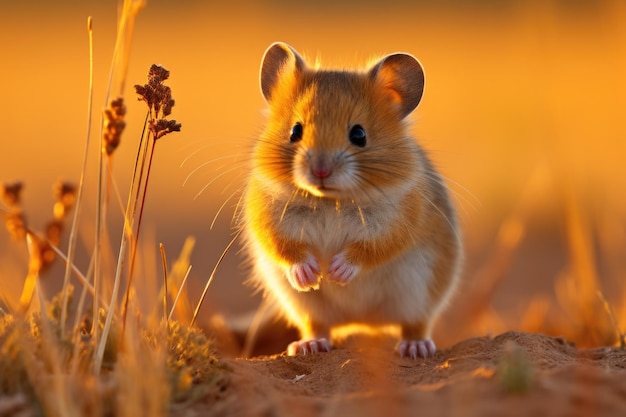A detailed photograph captures a small rodent—possibly a mouse or a hamster—against a warm, sunny backdrop. The creature stands alert on its hind legs on light-colored sand that blends into a blurred brown ground. Illuminated by sunlight, its orange-colored face is framed by beady black eyes, delicate black whiskers, and small, brownish ears. The rodent's light pink paws and feet, along with a white patch on its chest and around its nose, add contrast to its overall appearance. The ears appear somewhat flimsy, adding to its delicate demeanor. The background radiates an orange-yellow gradient from the sunlight, enriching the scene’s warm ambiance. To the left of the rodent, there are scattered dried grasses reaching upwards, intertwined with light reddish flowers emerging from the sandy ground, enhancing the scene's natural setting. The rodent's expression conveys a sense of alertness or concern, making the viewer ponder its thoughts in this evocative outdoor scene.